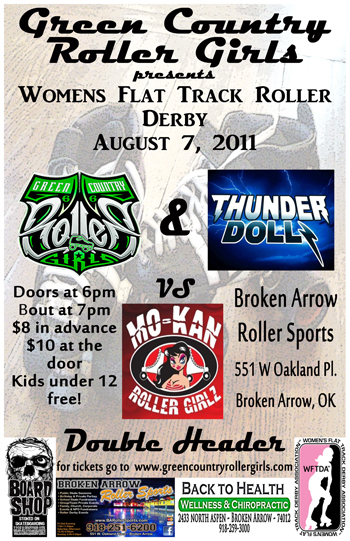This full-color advertisement poster for the Green Country Roller Girls presents a Women's Flat Track Roller Derby event that took place on August 7, 2011. The top of the poster features text in thick black cursive font stating "Green Country Roller Girls Presents" followed by "Women's Flat Track Roller Derby" in a standard capital letter font. Below this main heading, three logos are displayed: one green and silver crest for the Green Country Roller Girls, a logo with a black background and blue neon lightning for the Thunderdolls, and another red logo for the Mocan Roller Girls. 

On the left side of the red logo, the text reads: "Doors at 6pm, Bout at 7pm, $8 in advance, $10 at the door, Kids under 12 free." On the right side, the details include the venue: "Broken Arrow Roller Sports, 551W Oakland, PL, Broken Arrow, OK." Beneath the red logo, it also mentions "Double Header" and directs viewers to GreenCountryRollerGirls.com. Sponsored by Back to Health Wellness and Chiropractic and The Board Shop, additional intricate details and images, including a background with slightly blurred shoes on a ground floor, make up the bottom part of the poster.